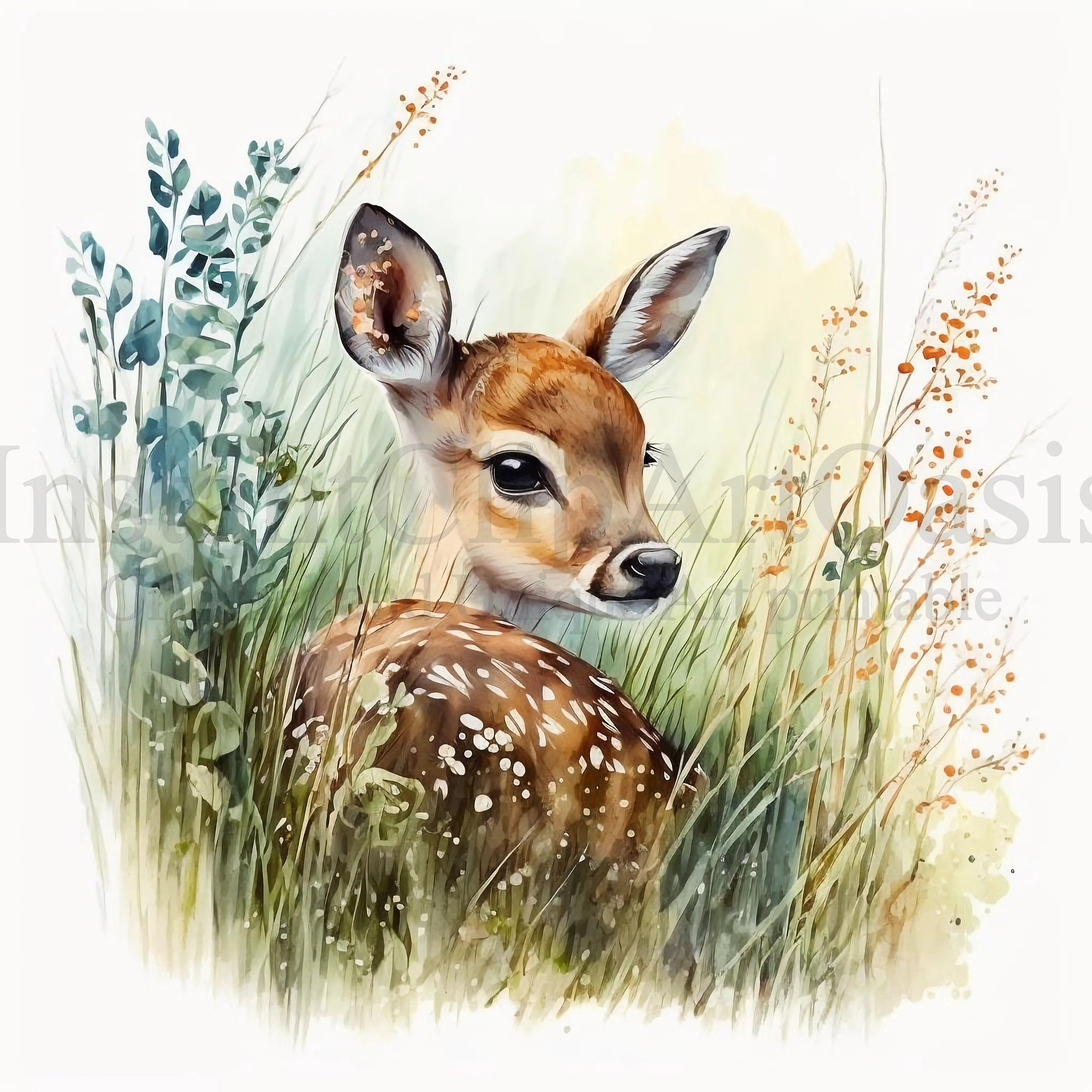This is a detailed watercolor painting of a baby deer, resembling Bambi, standing in the middle of a meadow. The light brown fawn, adorned with delicate white spots, has large, expressive eyes, a small black nose, and long eyelashes. Its ears, lined with short white fur inside, are perked upwards as it turns its head to the right, looking back at the viewer. The deer is depicted amidst tall green grass, which nearly reaches its head, with tall blue flowers on the left and peachy-orange blooms on the right. The background is a soft beige hue, adding to the gentle, serene atmosphere of the scene. The image has a watermark across it, bearing the partially visible text "clipart oasis."